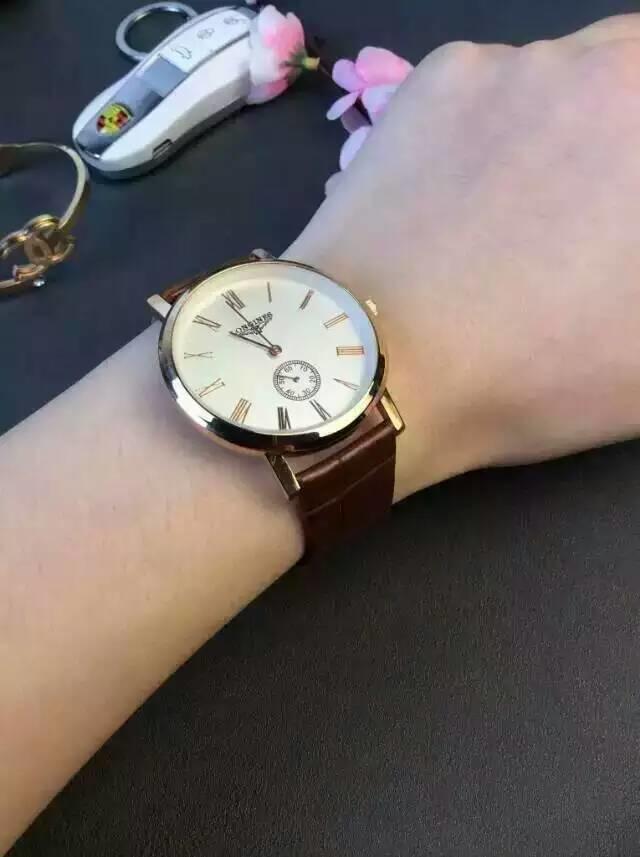In this color photograph, the focus is on a person's left wrist adorned with an elegant wristwatch. The watch features a dark brown leather strap and a white circular dial, outlined by a gold rim. The face of the watch displays Roman numerals, with the hands indicating the time as 11:59. A mini subdial, positioned at the six o'clock mark, showcases the second hand, distinguishing it from the main hour and minute hands. The manufacturer’s name, "LONGINES," is visible beneath the 12 o’clock mark. The watch’s long lugs contribute to its sophisticated appearance. 

In the background, the individual is holding a small pink flower. Adorning the wrist alongside the watch is a Chanel bracelet, identified by its interlocked C’s logo. The background also features a key fob bearing the Ferrari logo, adding a touch of luxury to the scene. The setting is against a predominately dark backdrop, with splashes of color from artificial pink flowers, creating a refined and tasteful composition.